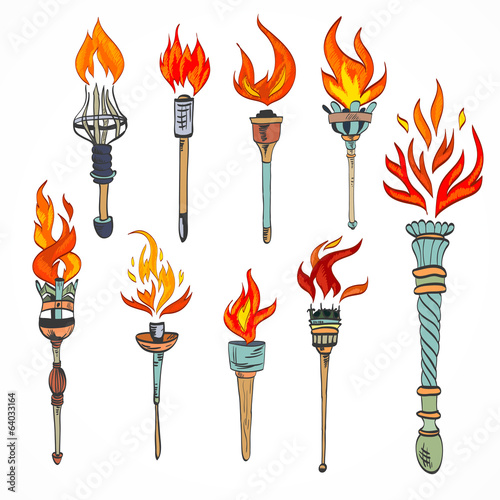The image depicts nine hand-drawn torches arranged in two rows against a backdrop with the watermark "Adobe Stock #64033164." The top row features four torches, each with distinct handle designs and varying flame styles in red, orange, or yellow hues. The bottom row displays five additional torches of diverse styles, handles, and lengths, with the one on the far right standing out as the largest. The torches exhibit a range of materials, including wood, metal, and dishes with spouts, characterized by intricate and ornate details. The primary colors used are greens, oranges, and blacks, complemented by some blue and brown shades on the handles. The background has a diagonal, watermarked "Adobe Stock" label in white, set against a darker grayish tone, with the text "Adobe stock" identifiable in black writing in the bottom left corner.